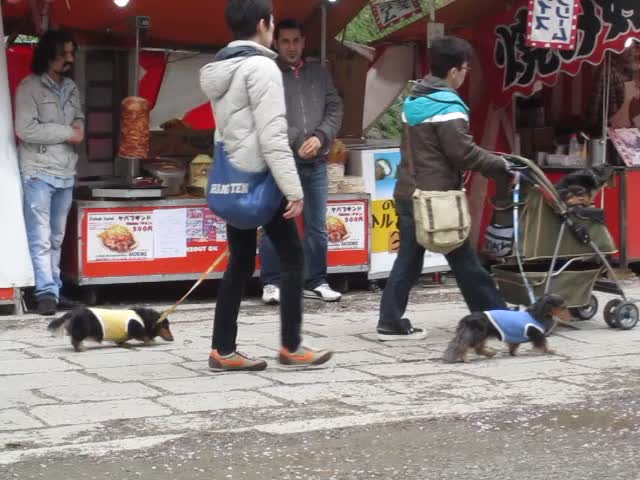In this vibrant outdoor market scene, a row of street vendors lines the background, one of which features a red tent with photographs of products on display at the front of their table. Among the vendors, a man in a tan top and jeans stands beside a cart showcasing a large meat skewer ready for slicing. The pathway in front of the stalls is comprised of rectangular stone pavers. Walking along this pathway are two individuals who appear to be of Asian descent, each accompanied by a dachshund. The person in the back left wears a white puffer jacket, black pants, and tan-black-orange sneakers, and carries a blue sling bag while walking a black dachshund with a yellow harness. In front of them, another person dressed in a brown jacket with a teal top section pushes an olive-green stroller. This person holds the leash of a long-haired black dachshund donning a blue harness while another dachshund peeks out from the stroller. The woman has short dark hair and wears jeans, completing her look with a brown bag. The overall scene captures a slice of everyday life in what looks like a bustling, culturally rich market area.